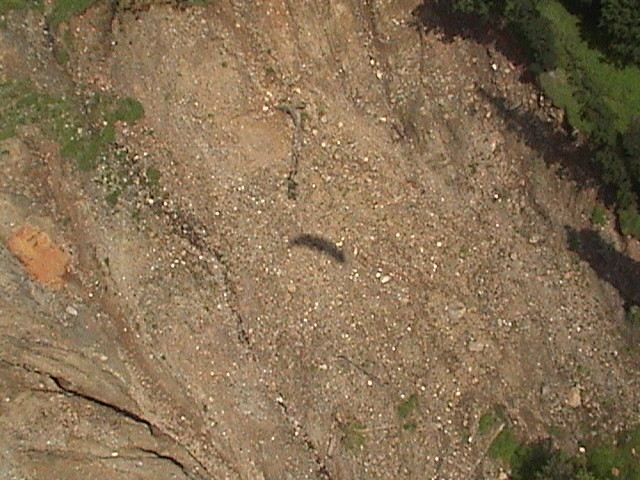The photograph captures an aerial view of a rugged, dirt-covered hillside, possibly part of a mountain, characterized primarily by its granular terrain made up of rocks and detritus. The landscape is largely devoid of lush vegetation, although patches of grass and trees can be found in the upper right and lower left corners of the image. The ground appears to be worn and fragmented, with visible signs of erosion possibly caused by recent rainfall, as indicated by the presence of mud and water-formed ravines cutting through the dirt. The terrain shows significant elevation changes, suggesting a slope or cliff face descending towards the upper right of the image. Central to the scene are two shadows that hint at an overhead perspective: one in the center resembling a parachute, indicating the photograph may have been taken by someone skydiving, and another to the right, reinforcing the idea of aerial or high-altitude photography. No people or animals are visible in the image, emphasizing the barren and desolate nature of the landscape.